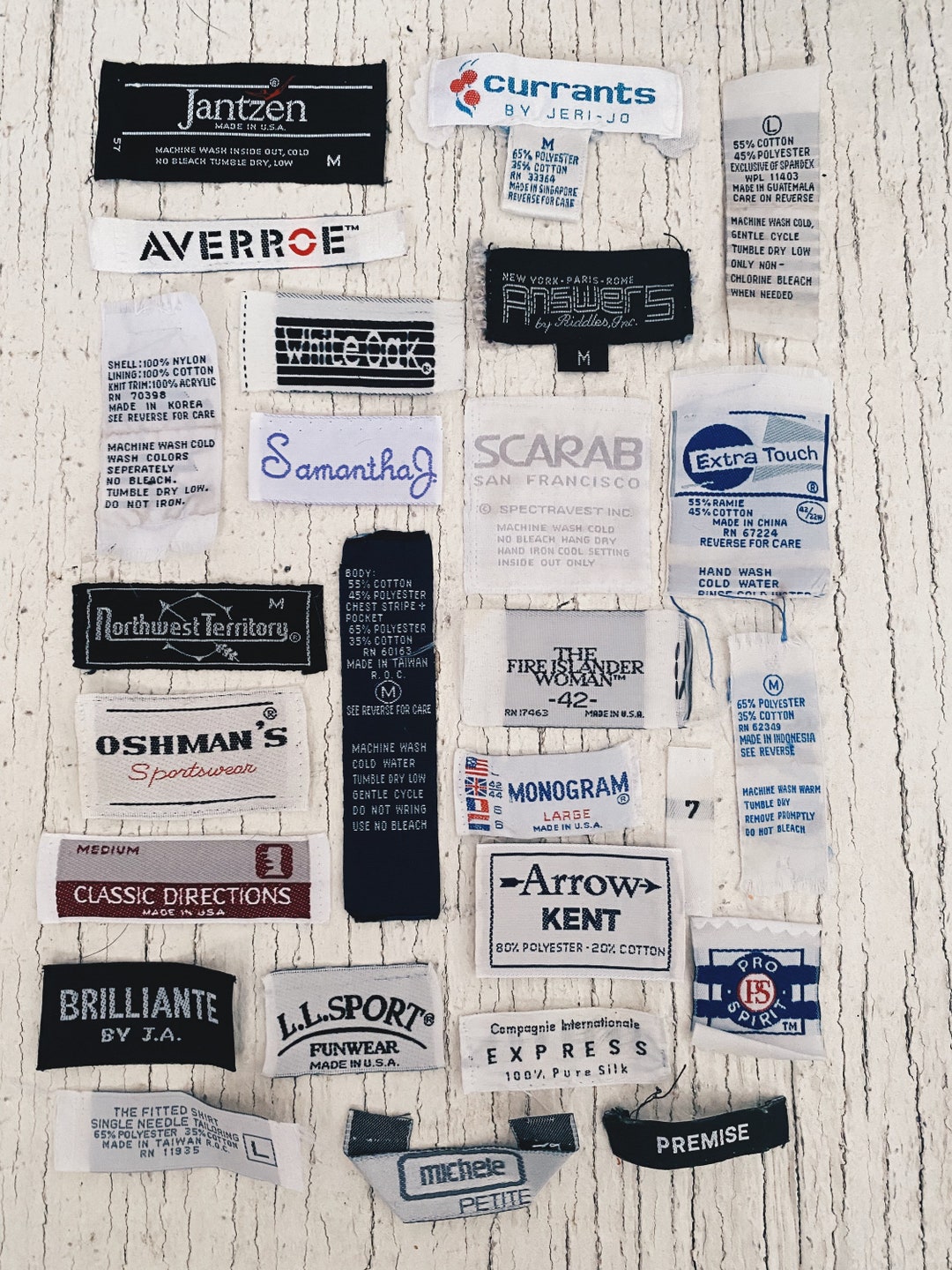Displayed against a weathered white-painted board are assorted fabric tags from clothing, neatly laid out in a rectangular photograph as if for a catalog. These tags, primarily rectangular or square in shape, vary in size and color—black and white being the most common. Brand names prominently featured include Janssen, Aero, LL Sport Funwear, Prentice, Pro Spirit, Currents, Avarochi, White Oak, Answers, Samantha J, Scarab San Francisco, Extra Touch, Northwest Territory, The Fire Islander Woman, Classic Directions, Arrow, Kent, Brilliant by J.A., Campaign International Express, Michelle Petit, and Premise. Some tags provide information on fabric composition, such as "65% polyester, 35% cotton," while others indicate garment care instructions like "machine wash warm, tumble dry, remove promptly, do not bleach." Sizes are also displayed, often marked with an "M" for medium. While seemingly random, these tags collectively offer an intriguing glimpse into the variety of clothing brands and manufacturing details.